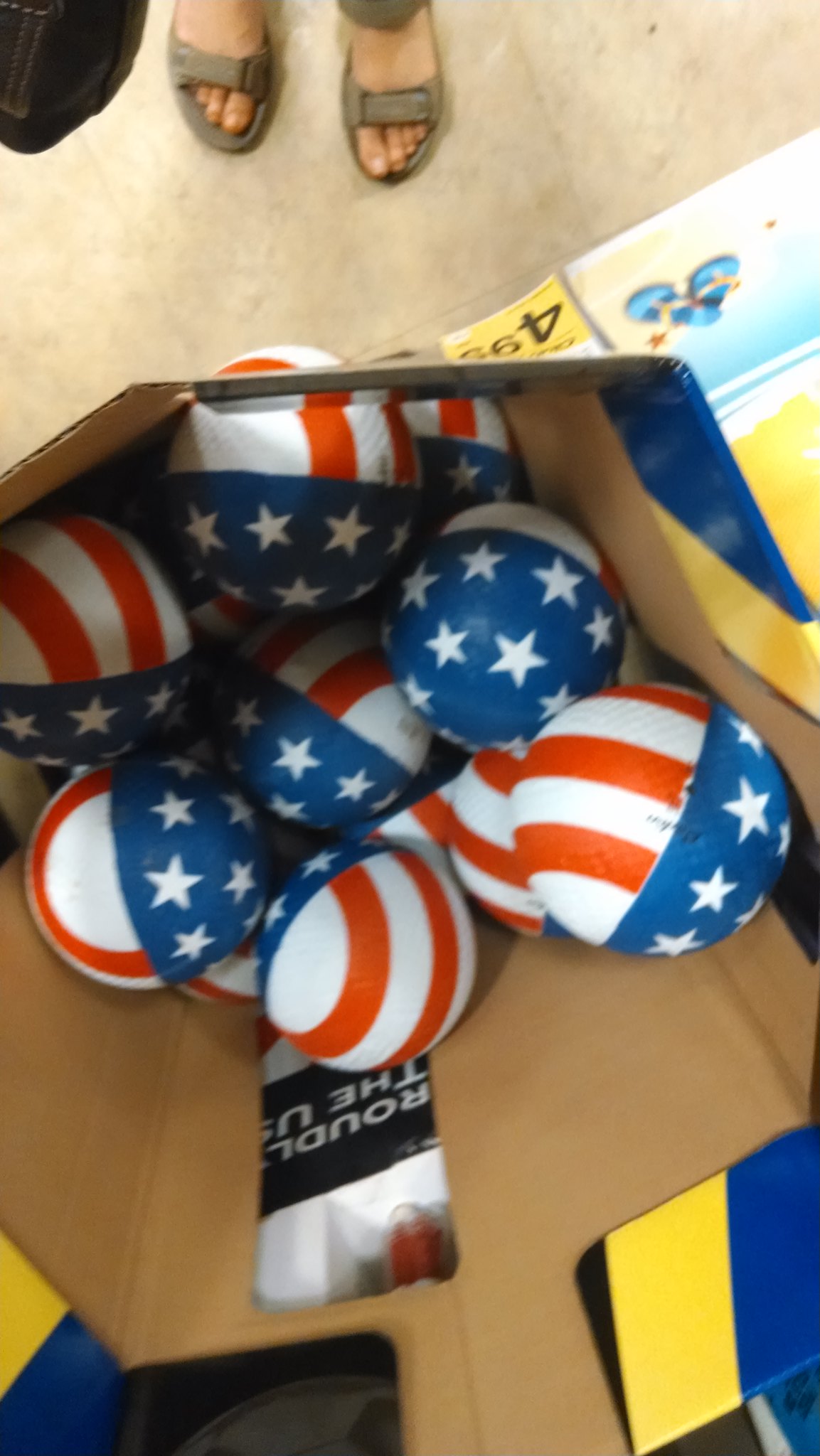The image depicts a store setting and is taken from an elevated perspective, looking downward. At the top of the image, part of a beige store floor is visible, along with the sandaled feet of a person, suggesting these are women's feet due to the presence of a bag typically carried by women. In the middle, a tall, blue and yellow cardboard box with folded-down corners contains several bouncy balls designed to resemble Captain America's shield. Each ball features red and white stripes on one side and a blue section with white stars on the other. The box itself has an octagonal shape and a noticeable hole on one edge.

Beneath the box, a rack holds flip-flops priced at $4.99, according to a small yellow sign. The display is a bit cluttered, with some text visible behind the box. However, the words are partially obscured, showing only fragments like "R-O-U-D-L, the, and U-S." The image includes additional signage around the display, contributing to the overall busy appearance of the scene. The photo is slightly blurry, adding a sense of casualness and hurriedness to the captured moment.